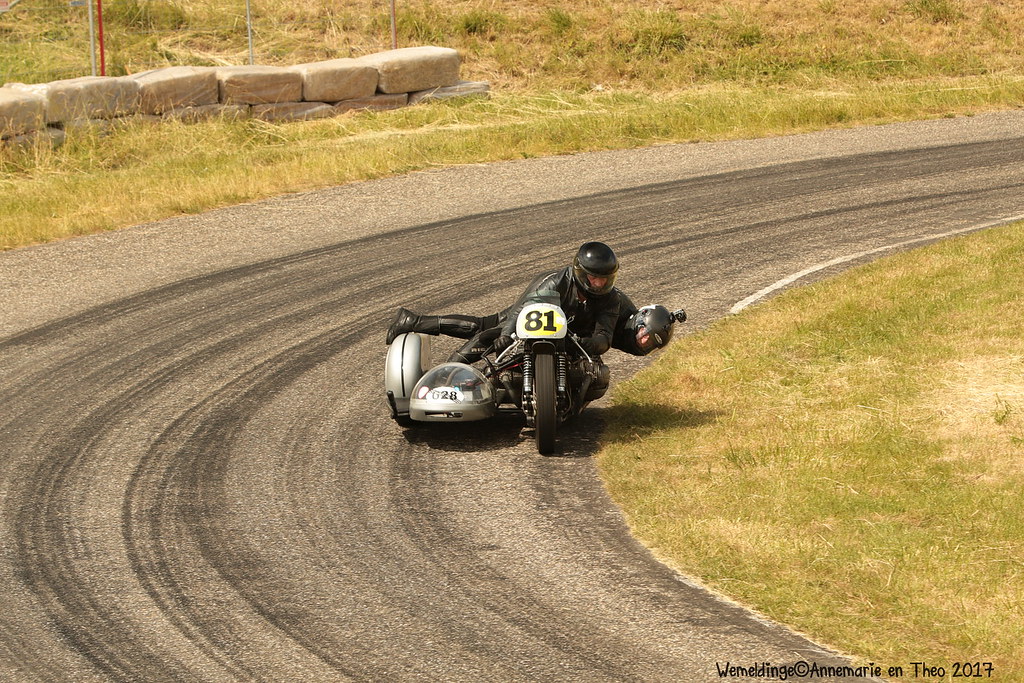In this image, two racers are navigating a sharp left-hand corner on a black and silver sidecar motorcycle on a worn dirt track, evidenced by the numerous tread marks visible. Both racers are dressed in black leather suits and black helmets for protection. The rider operates the motorcycle while the passenger leans deeply into the curve from the sidecar, appearing to struggle slightly with the angle. The motorcycle prominently features the number 81 at the front, with a small compartment to the side marked with the number 028. Surrounding the track are stacks of hay bales to the left and a mix of green and yellow grass on both the inside and outside of the track. In the upper left-hand corner, a wall of rocks is visible, providing a rugged backdrop under the sunny sky. The bottom right-hand corner of the picture includes the text, "W.E. Melding E. Anne-Marie E.N. Theo 2017."